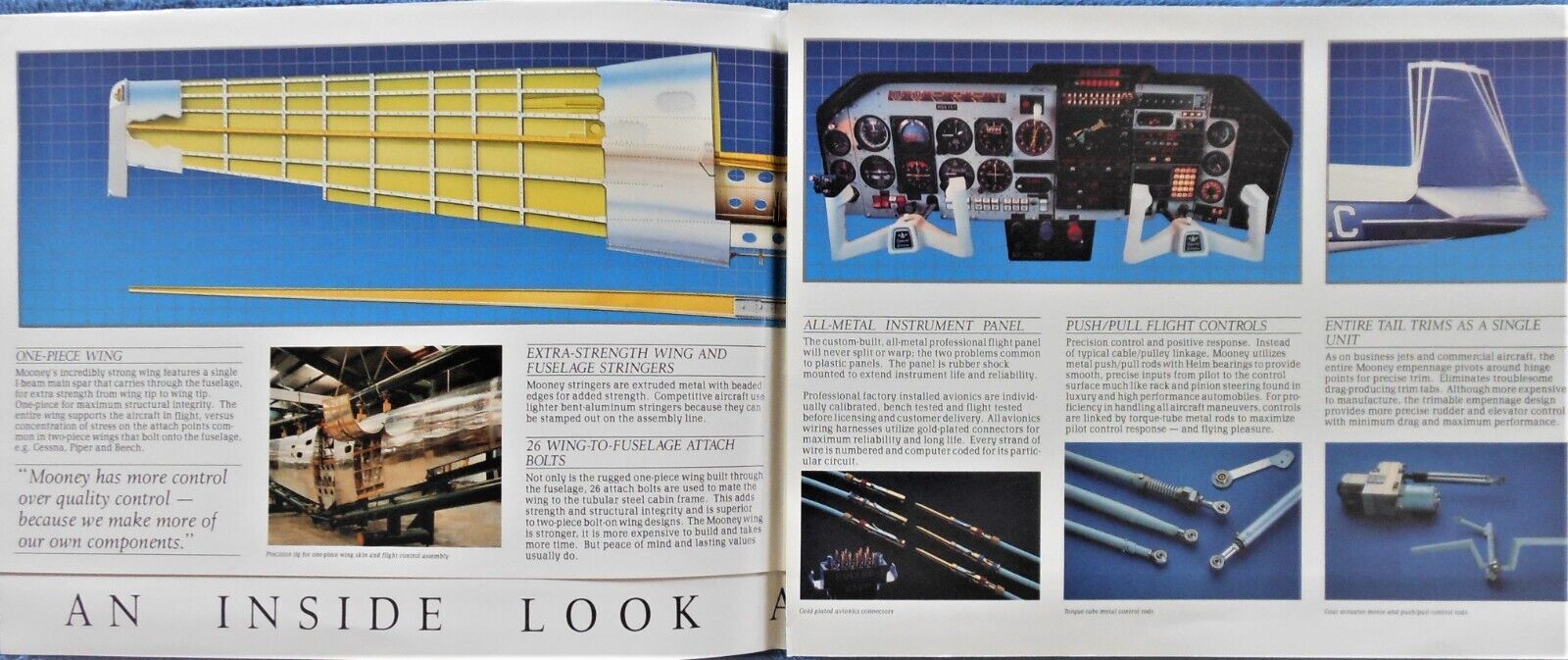The image depicts a wide, rectangular photograph of an open book, showing both the left and right pages. The left page features a detailed image with a blue and white grid pattern, revealing an inside look at various airplane components, particularly a section of an aircraft's fuselage with a yellow metal gridded structure. Below this image are paragraphs of text explaining the components. Bold text at the bottom of the left page reads "An Inside Look."

On the right page, the top half of the space displays a mock-up image of a plane's cockpit, showcasing an all-metal instrument panel. Adjacent to this is a picture of a plane's tail fin. The lower half of the right page contains three detailed images labeled with descriptions: "All Metal Instrument Panel," "Push-Pull Flight Controls," and "Entire Tail Trims as a Single Unit," each representing different parts of the airplane. This book page appears to be focused on explaining various mechanical aspects and components related to flight mechanics or a flight simulator, featuring both instructional text and detailed photographic elements.